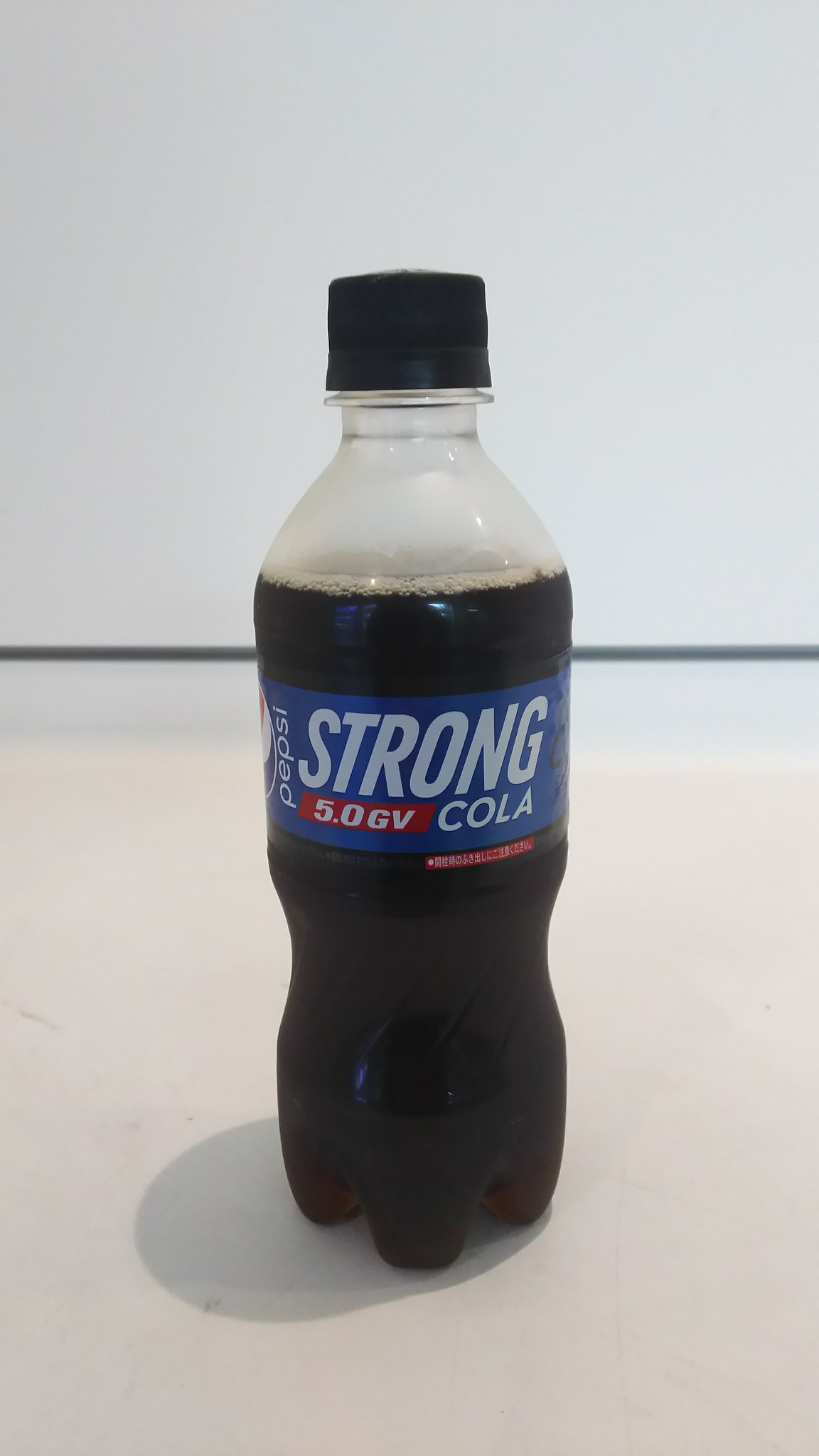The image features a close-up of a plastic Pepsi Strong Cola bottle, prominently displayed on a pale blue surface with a black horizontal line running through the background. The bottle is transparent, revealing a dark, cola-colored liquid filled all the way up. It has a black screw cap and a distinct blue label encircling the bottle. On the left side of the label, "Pepsi" is vertically inscribed in white text alongside the iconic red, white, and blue logo. The center of the label boasts "Strong" in large, bold white letters, followed by "Cola" and a small red ribbon marking "5.0 GV." The design and presentation of the label clearly differentiate this as a Pepsi Strong Cola variant.